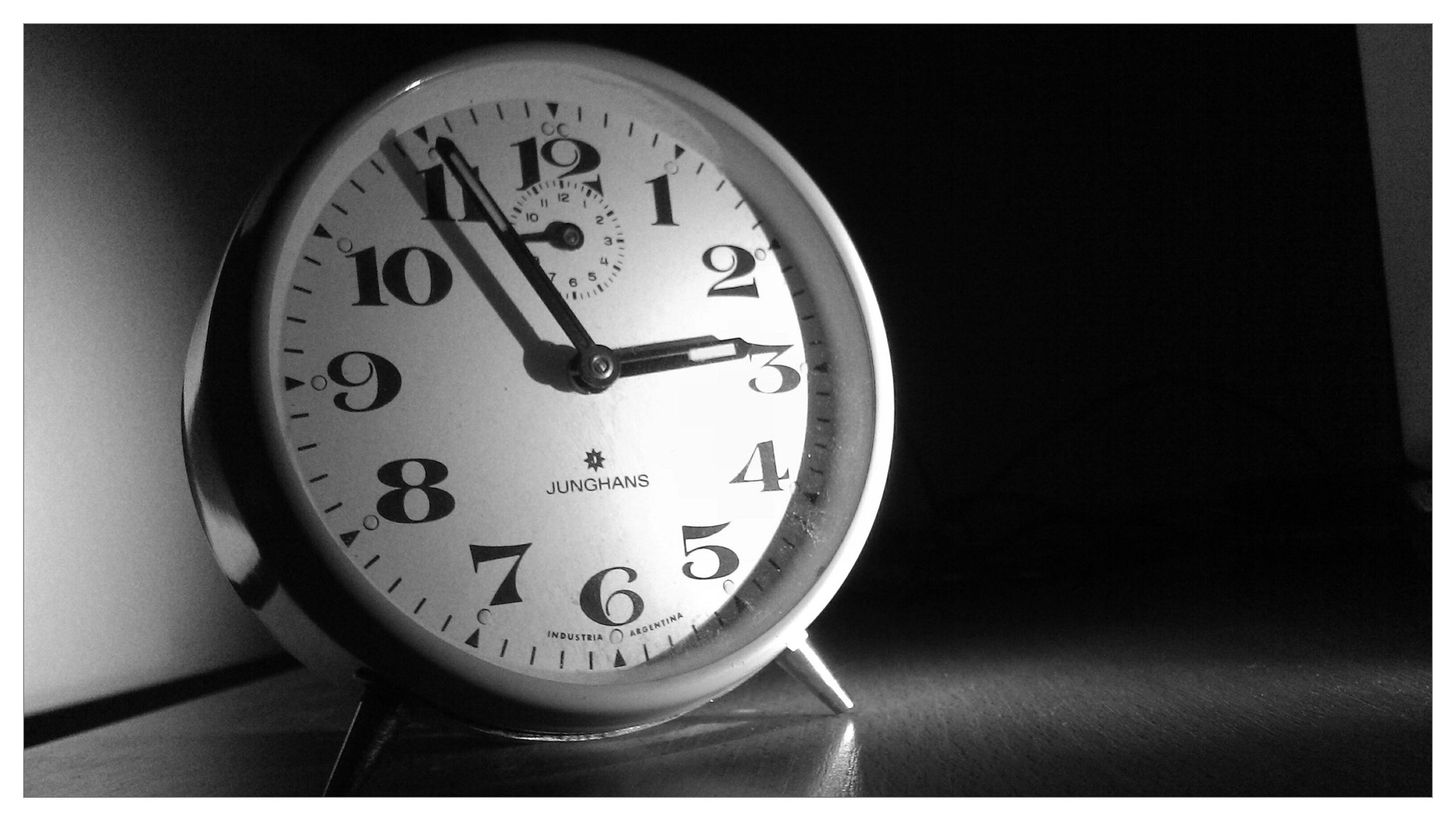This photograph captures a small, white circular alarm clock set against an indistinct, artistically blurred background. The clock features bold black numbers and tick marks, with its hands indicating the time as 2:54. The right side of the image is more shadowed, creating a subtle contrast that highlights the alarm clock's form. The clock is placed on a textured surface resembling faux wood, adding an element of rustic charm to the composition. The overall lighting accentuates the clock, making it the focal point of this clean and minimalist scene.